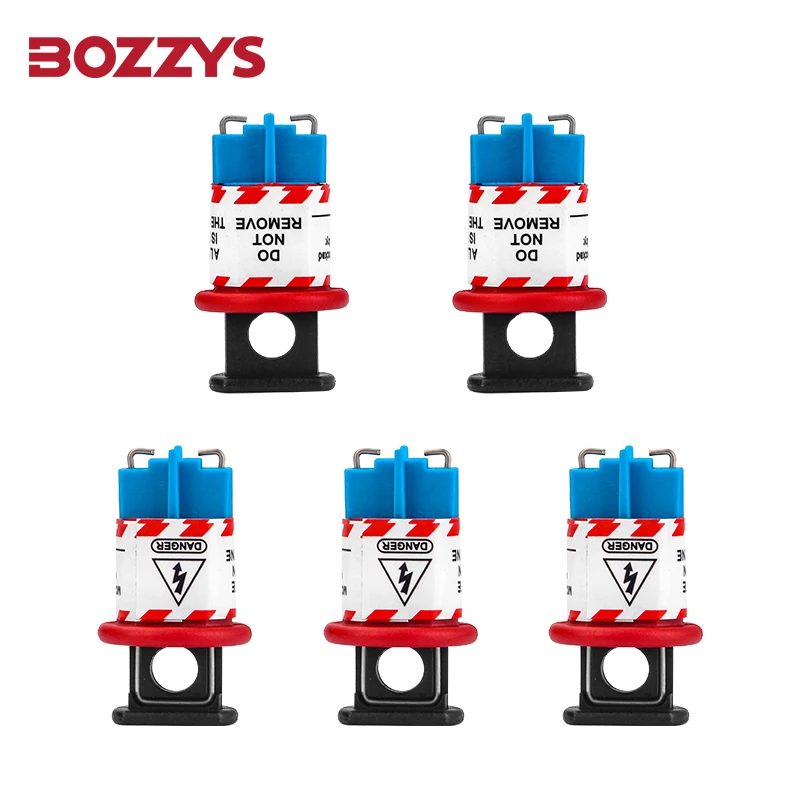This image features a collection of five identical electrical components arranged against a white background. In the top right corner, the word "BOZZYS" is prominently displayed in dark red, boxy text. Each component consists of a blue rectangular base with metal prongs protruding from the top, half-covered by a white sticker adorned with red and white zigzag lines. The two components in the top row display the warning "DO NOT REMOVE" in black font, while the three in the bottom row bear the word "DANGER" along with a black triangle icon featuring a lightning bolt, indicating high voltage risk. At the bottom of each blue rectangle, a red horizontal tab extends perpendicularly, supported by a black pedestal with a central hole. Notably, all five components appear upside down in the image.